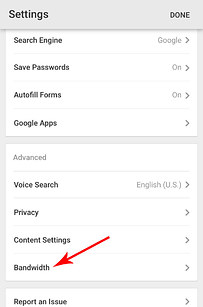This screenshot shows the settings page of a web browser, likely Google Chrome, featuring a clean and minimalist design with a gray and white color scheme. In the upper right corner, there's a "Done" button. The page is organized with multiple clickable categories: 

- **Search Engine**: Currently set to Google
- **Save Passwords**: Enabled
- **Autofill Forms**: Enabled
- **Google Apps**: A dedicated section
- **Advanced Section**: Several detailed settings available

Within the advanced settings, categories like **Voice Search** are set to English (US), along with other settings for **Privacy**, **Content Settings**, and **Bandwidth**. Notably, there's a red diagonal arrow pointing towards the bandwidth section, highlighting its importance. Additionally, there's a **Report an Issue** category. The overall layout is basic yet functional, tailored for ease of navigation and user-friendliness.